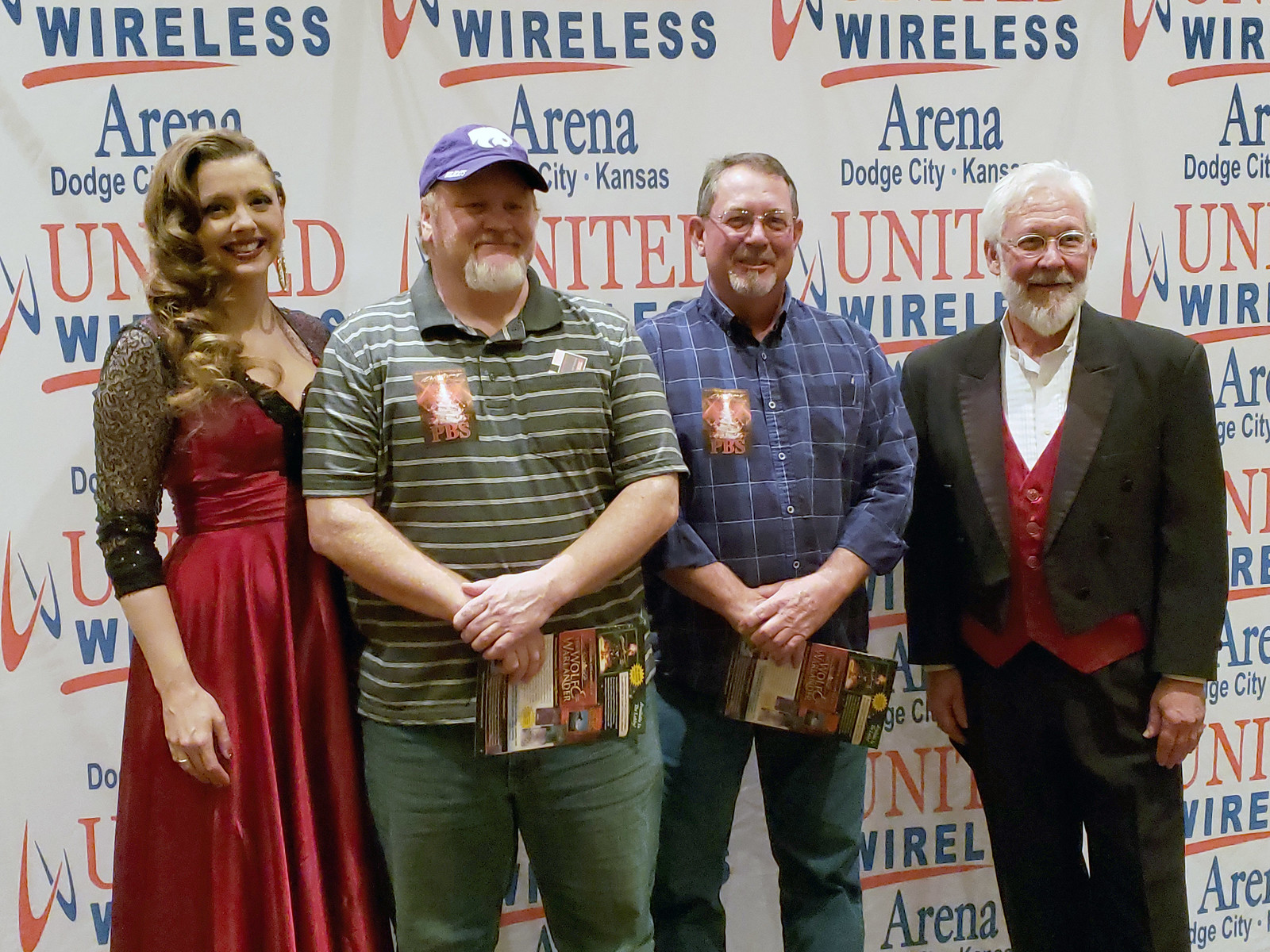This color photograph features four adults standing on a stage, all facing the camera. From left to right, the first individual is a blonde woman, elegantly dressed in a red and black formal gown, radiating a warm smile. To her right, the second person is a man holding a booklet, also smiling. He is casually dressed in blue jeans and a green and white polo shirt, topped with a blue baseball cap. The third man, similarly dressed in blue jeans, is wearing a blue and black plaid button-down shirt. He has short hair and a gray beard, giving off a friendly demeanor. The last person on the far right is dressed in a black tuxedo-like suit with a red vest, harmonizing with the woman's outfit on the far left. His formal attire suggests he might be one of the key figures of the event.

The woman in the elegant dress and the man in the tuxedo bookend the group, possibly hinting at their roles as officiants or hosts of what seems to be an award ceremony. The two casually dressed men in the middle, holding a booklet and standing in more relaxed postures, appear to be the recipients of some awards or recognition. The carefully coordinated outfits and the stage setting imply a significant event, possibly celebrating achievements or milestones.